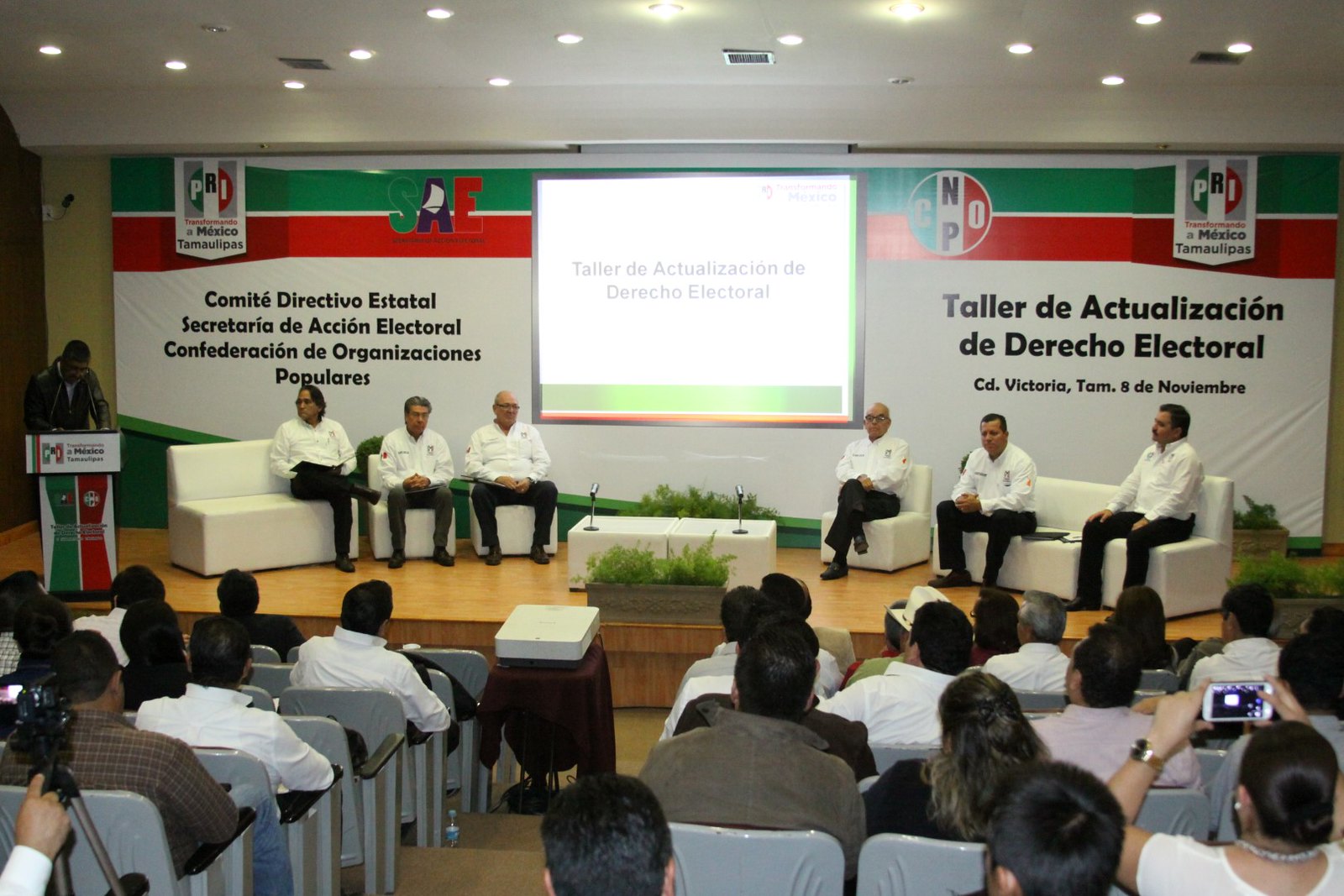In this photograph, we see a conference taking place in an auditorium-like room. The stage is slightly elevated from the audience and features six men seated on a variety of white sofas and chairs. These men, dressed in black pants and white dress shirts with no ties, are divided into two groups of three on either side of a small central table equipped with microphones.

To the far right of the stage, a person stands at a podium. This podium appears simple, white in color, and adorned with logos and emblems in green, red, and white. Behind this person is a large banner featuring text in Spanish, which includes words such as "Comité Directivo Estatal," "Secretaría de Acción Electoral," and "Conferencia de Organización de Colonias Populares." These phrases suggest that the event is related to electoral activities in a Spanish-speaking country, possibly Mexico, as hinted by the word "Mexico" on the banner.

A bright screen in the middle of the background displays a slideshow titled "Taller de Actualización de Derecho Electoral," although the specific details of the slideshow are not clearly visible. The background also includes several emblems labeled "PRI" and "NPO."

The audience comprises individuals, mostly men dressed in white shirts, among whom some wear jackets. One can notice a person taking pictures and another woman using her phone, possibly to record the event. A projector in the center of the audience area beams the slideshow onto the screen on stage. A decorative plant is situated at the front of the stage, adding a touch of greenery to the setting.